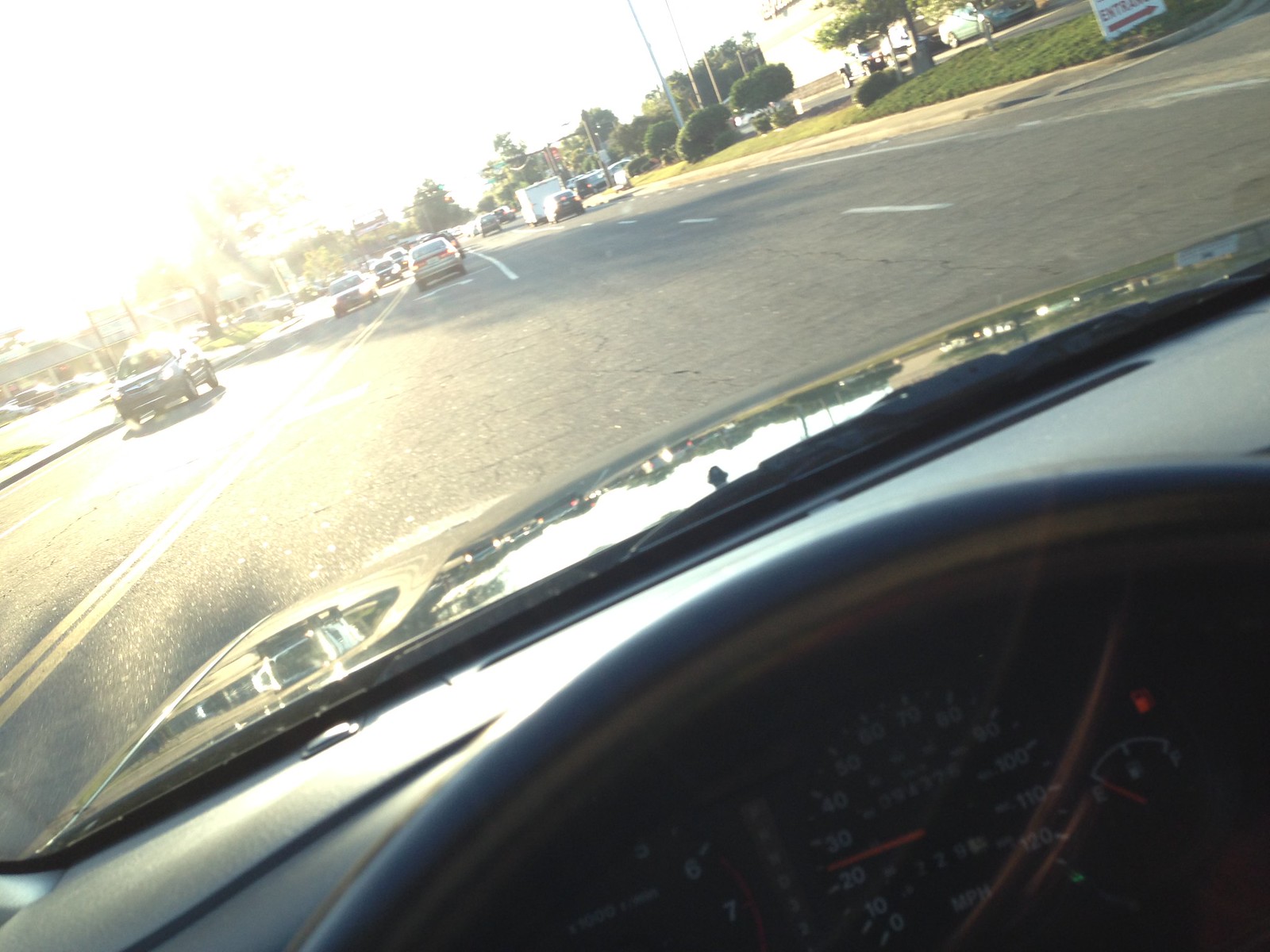Captured from inside a vehicle, this outdoor photograph showcases a sunny street scene viewed through the front windshield. The dashboard is partially visible, indicating an empty gas tank and a speed of approximately 25 miles per hour. The vehicle is positioned in the left lane, preparing to enter the left turn lane. Despite the bright sunlight causing significant glare on the street, cars in the opposite direction have their headlights on, an unusual sight. Ahead, other vehicles, including a box truck, are visible. The background is adorned with buildings and trees, enveloped in the sunny ambiance, further emphasizing the sun's strong presence.